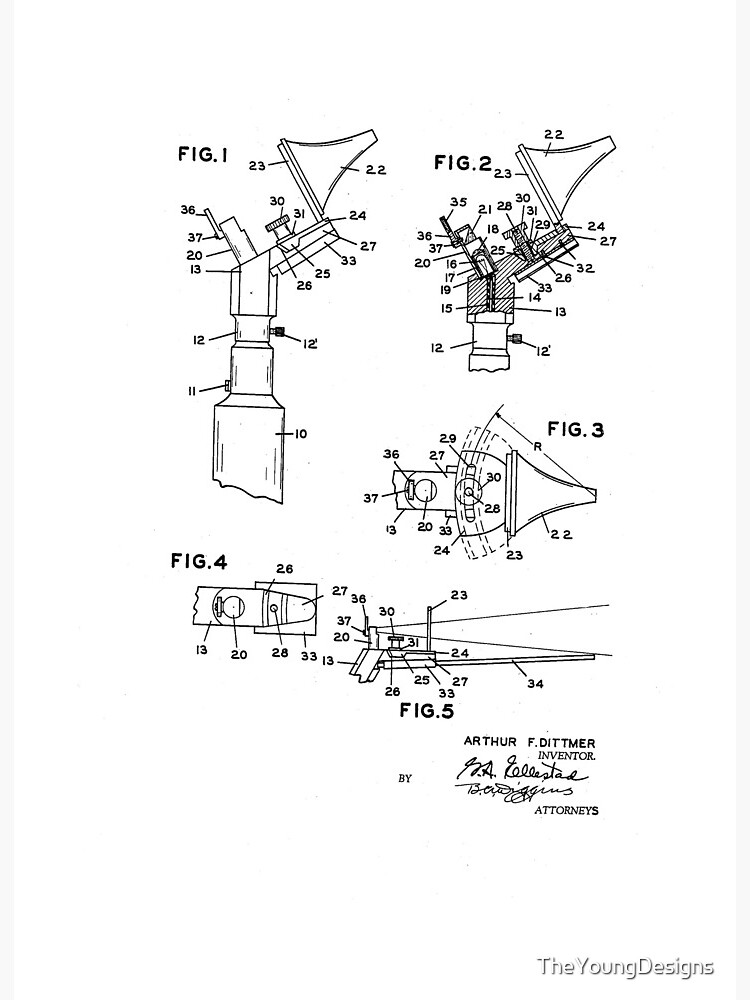This detailed drawing is a diagram likely illustrating the assembly or components of an invention, typical of a manual or technical textbook. Set against a white background, the black line sketches depict five distinct figures, each annotated with numerous intricate numbers corresponding to different parts. Figure 1, located at the top left, is long and narrow, featuring a triangle off to the left. Figure 2 sits to the right of Figure 1, similar in shape but slightly smaller. Below Figure 2, Figure 3 is horizontally oriented. Figure 4, positioned in the bottom left, appears small and ambiguous, while Figure 5, the final figure, contains an array of lines and numbers that make it complex to interpret. All figures are labeled with abbreviated identifiers such as "Fig. 1," "Fig. 2," through "Fig. 5." Along the bottom of the diagram, a watermark reads "The Young Designs," and higher up, a signature notes "Arthur F. Dittmer, Inventor," followed by another signature and the word "Attorneys."